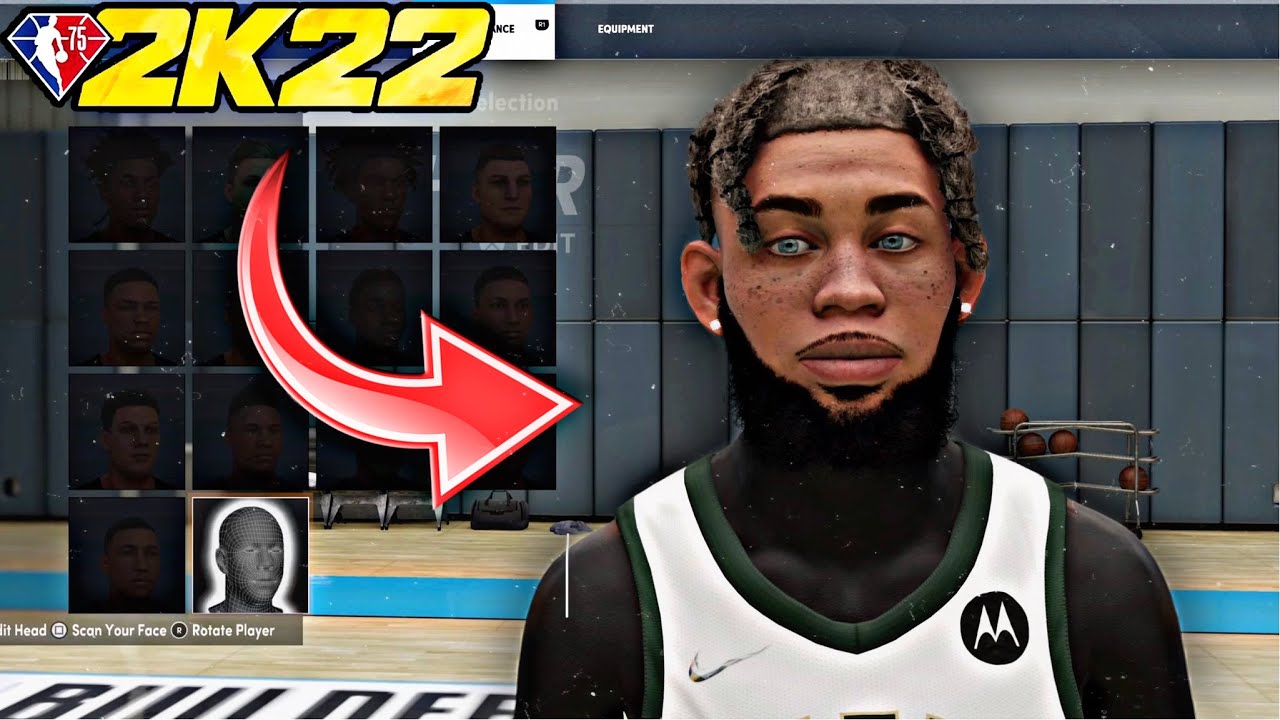This image is a screenshot from the NBA video game "NBA 2K22," as indicated by the game title prominently displayed in yellow text in the upper left-hand corner. In this corner, there is also a diamond-shaped icon featuring the silhouette of an NBA player in action, clutching a basketball. The background incorporates navy areas on the left and red on the right, with the number "75" shown in white next to the silhouette, hinting at the game's celebration of the NBA's 75th anniversary.

In the main focus of the image, there is an African-American player wearing a white jersey trimmed in green. The player's complexion is notably dark at the bottom, transitioning to a brownish hue towards his face. His facial features include blue eyes, light facial hair above the lip forming a mustache, a slight goatee beneath the lip, and a fuller beard. Additionally, he is adorned with white earrings and has visible freckles on his face.

A red arrow curves down from the "2K22" text and points directly at this player, highlighting him as the central subject of the image.